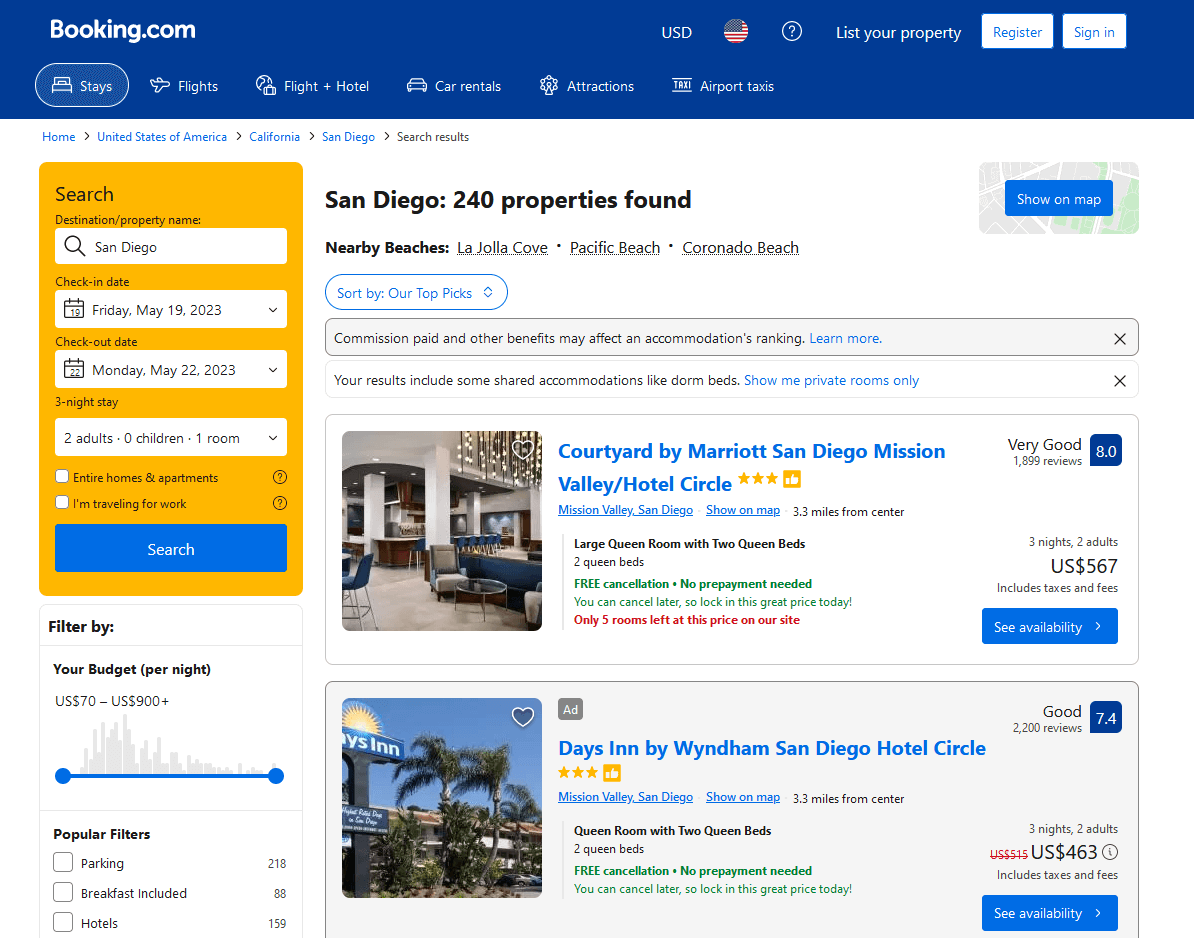The screenshot showcases the homepage of the website Booking.com. In the upper left-hand corner of the screen, the Booking.com logo is prominently displayed within an extensive blue banner that stretches across the top of the website. Adjacent to the logo, various functional tabs are visible including currency settings labeled 'USD', and an icon of a question mark encircled, which provides more information. The banner also offers options to list a property, register for a new account, or sign in for existing users.

Beneath the blue banner, several navigation tabs are available, each leading to different services: 'Stays', 'Flights', 'Flight + Hotel', 'Car Rentals', 'Attractions', and 'Airport Taxis'. Scrolling further down, a bright gold search box stands out, designed for users to input their destination or property name. Underneath this, fields are provided for check-in and check-out dates, specified for a three-night stay. Additional fields ask for the number of adults, children, and rooms required. There are also options to indicate whether the search is for an entire home or apartment, or if the user is traveling for work.

In the middle section of the page, some example properties are showcased, such as the Courtyard by Marriott San Diego and the Days Inn in San Diego, offering a preview of available accommodations.